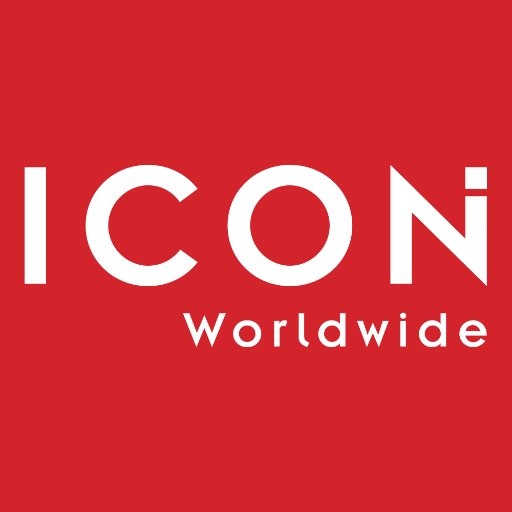The image features a bold, striking logo with a red-orange background and white lettering. Dominating the center are large, capital letters spelling "ICON," where the top right part of the 'N' has a distinctive dot-like break. Below "ICON," offset slightly to the right, the word "Worldwide" is displayed in smaller font, with a capital 'W' followed by lowercase letters. The layout appears meticulously balanced, with "ICON" centered and ample spacing creating a division that visually splits the image into thirds. The overall design suggests a corporate identity, likely for a company named Icon Worldwide, with a clean and easy-to-read, though slightly unconventional, font style.